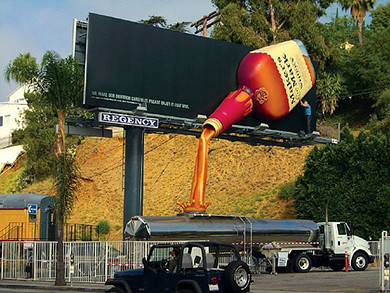The photograph captures a rectangular scene with a large billboard positioned towards the upper section. The billboard itself features a dramatic black background, prominently showcasing a striking 3D whiskey bottle with an attention-grabbing design. The whiskey bottle, part of a clever advertisement, appears to be pouring its contents downward. The bottle's large white label clearly reads "Maker's Mark," emphasizing the brand.

Beneath this creative display, a sizeable tanker truck is strategically placed. The illusion is crafted with a plastic representation of pouring liquid that seamlessly connects to the truck's spout, ingeniously designed to make it appear as though the whiskey is being funneled directly into the truck’s trailer. This imaginative setup on the billboard combines visual appeal with smart marketing, creating a memorable and eye-catching advertisement for Maker's Mark whiskey.